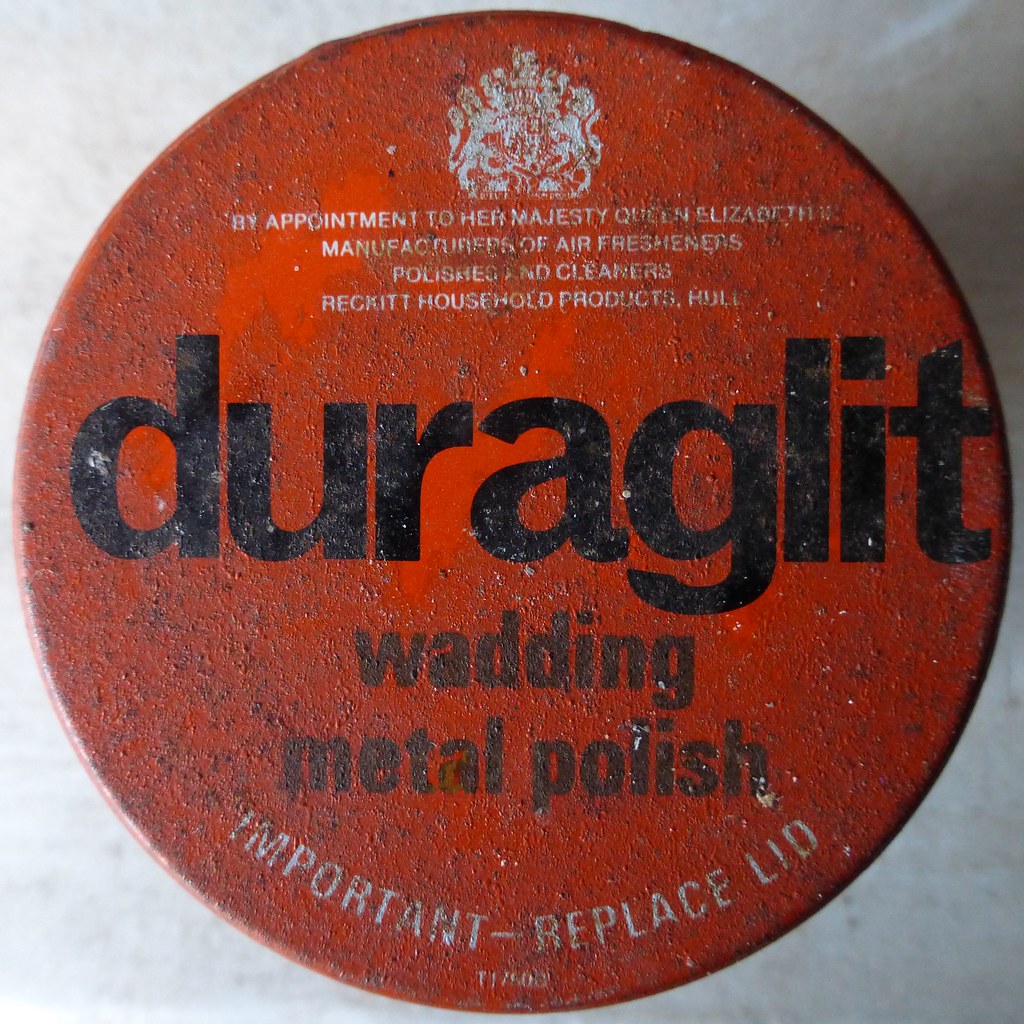The focal point of the image is an old, round, red lid, its color now faded to a burnt orange. This lid, which appears to be from a tin, features a roughly textured, worn surface. Dominating the central position of the picture, the lid is adorned with various texts and a logo that indicate its former grandeur. 

At the top center, there is a white crest, beneath which the text reads: "By appointment to Her Majesty Queen Elizabeth, manufacturers of air fresheners, polishes, and cleaners, Beckett Household Products, Hull." Central to the lid, in bold black letters, it reads: "Dura Glit, Wadding Metal Polish." Additionally, smaller white text at the bottom of the lid stresses: "Important, replace lid."

The cumulative elements of the textual and visual details emphasize the age and historical value of the lid, capturing the specific branding and royal endorsement, while the faded and worn state suggests extensive use over time.